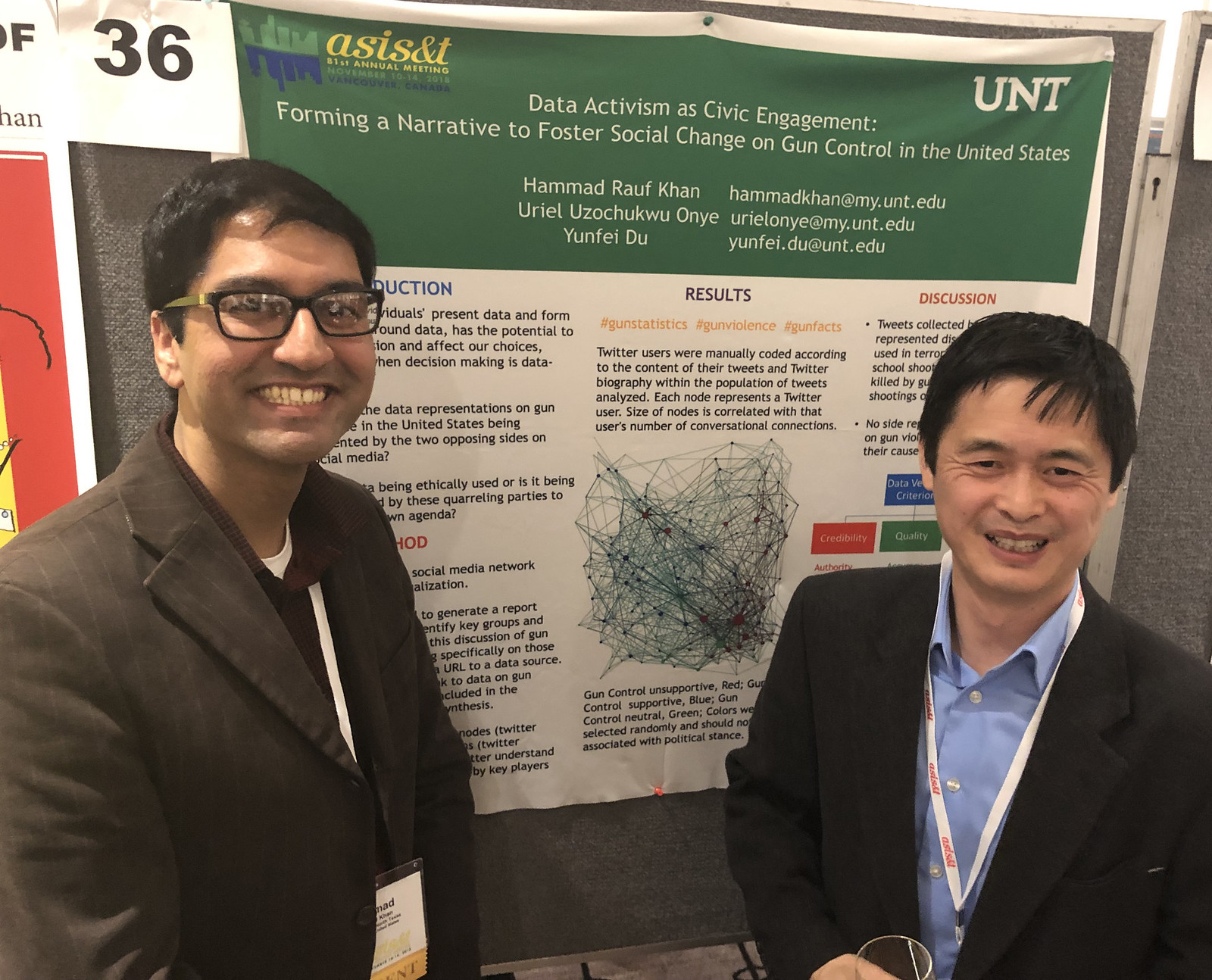In the image, there are two men standing in front of a grey fabric bulletin board with a poster attached to it. The man on the left, who appears to be of Muslim descent, is smiling and wearing black eyeglasses. He has short black hair and is dressed in a brown suit with white stripes, complemented by a purple polo shirt underneath. A name tag is hanging on his chest. The man on the right, who looks Asian and is shorter, is also smiling. He has short black hair and is dressed in a black suit with a light blue shirt. Although his name tag is partially obscured, the white supporting line is visible attached to his leg. 

The poster behind them is titled "Data Activism as Civic Engagement: Forming a Narrative to Foster Social Change on Gun Control in the United States" and includes names like Hamad Raf Khan, Yaryel Uzochukwu Onye, and Yufei Du. The text on the poster discusses the analysis of Twitter data related to gun control and illustrates the findings with hashtags such as #gunstatistics, #gunviolence, and #gunfacts. The nodes on the poster represent Twitter users, with their sizes correlating to the number of their conversational connections. They appear to be at a conference, indicated by the number 36 attached to the sign, highlighting their data activism work and the friendly, approachable nature of the presenters.